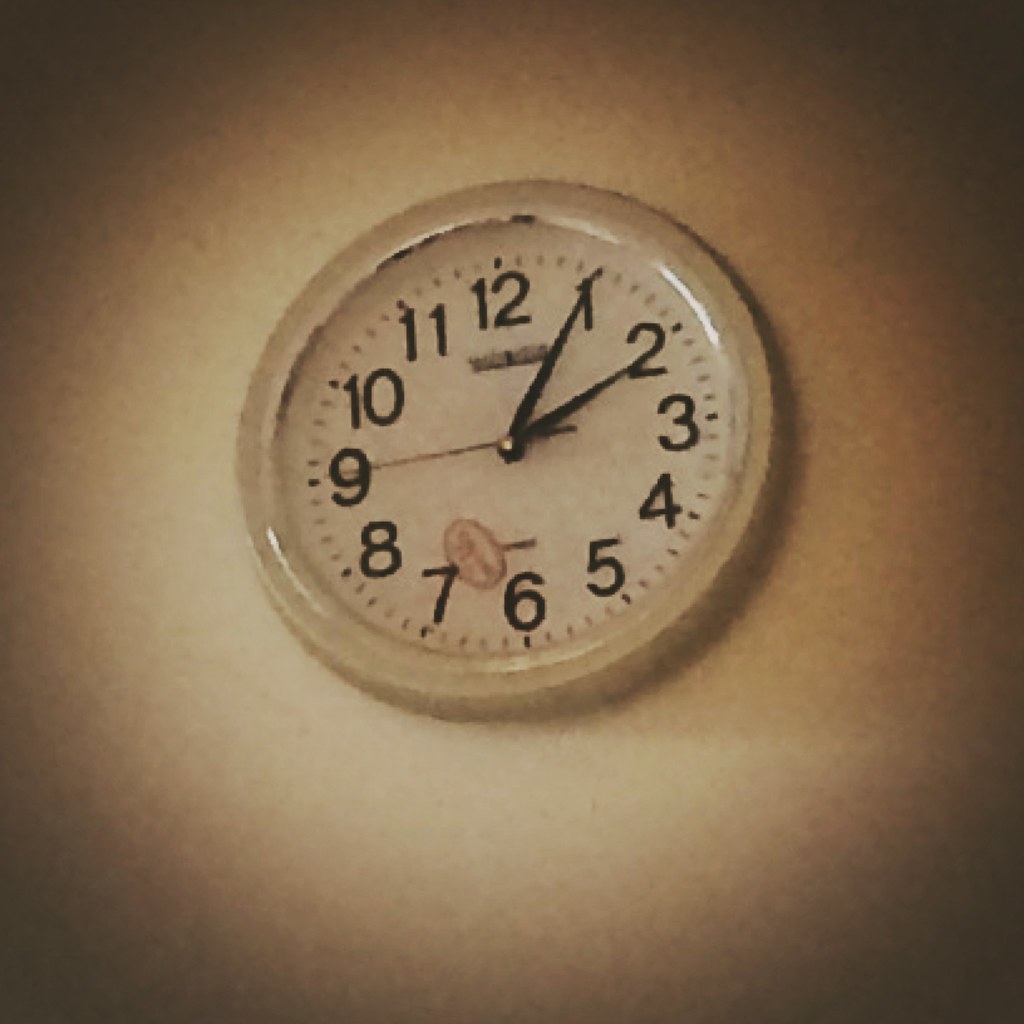This image features a slightly blurry photograph of a basic, old-fashioned white clock mounted on a wall. The clock, which appears worn and chipped at the edges, has a circular shape framed by a white metal border. Its face is also white, adorned with traditional black numbers ranging from 1 to 12. The clock displays the time as 2:05, with the small hand just past the 2 and the large hand on the 1. The red second hand is pointing to the 9, covering 45 seconds. An oval-shaped decal, featuring a red streak, is positioned above the number 7, partially obstructing it. The background is a plain wall, described as either white or beige, with the image showing a shadow cast on the right side and darker corners, adding a vignette effect.